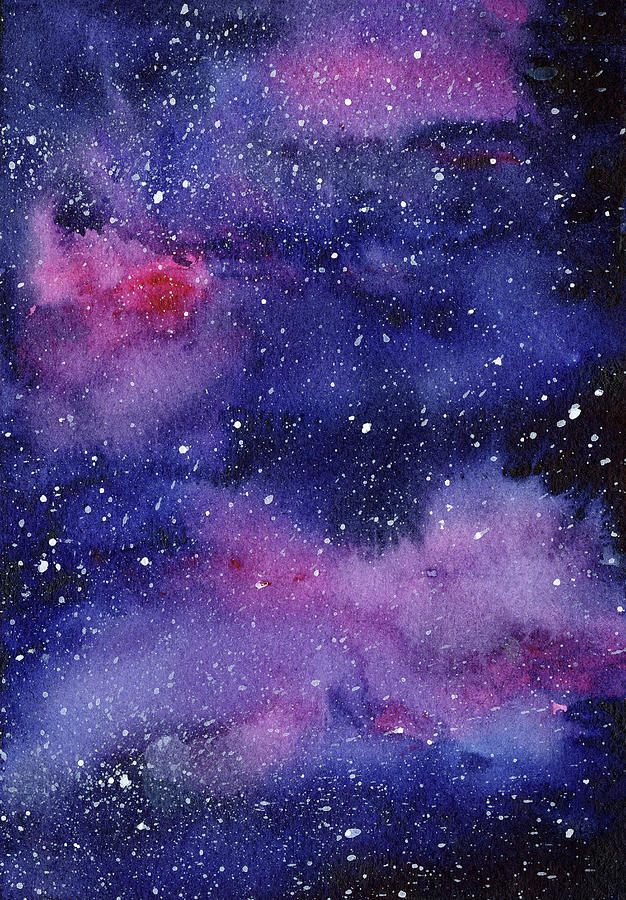This image captures a stunning, close-up view of a celestial scene, possibly a photograph from a telescope. The background is predominantly dark black, especially more pronounced in the corners, creating a vast and expansive night sky. Scattered throughout this black backdrop are thousands of tiny, white specks and flecks, representing distant stars and galaxies. 

The foreground is dominated by ethereal clouds of cosmic dust and gas, rendered in a mesmerizing palette of colors. These colors transition seamlessly from deep blue to vibrant pink, lighter purple, and shades of reddish-white. The colors are wispy and faint, allowing the dark sky to peek through in places, adding depth and texture to the scene. 

One notable feature is a bright pink spot towards the left of the image, contrasting with a predominantly purple area at the top center. The entire composition, with its sporadic, painted-like appearance, evokes a sense of grandeur and beauty inherent in the cosmos. The interplay of light and color, against the backdrop of the infinite night sky, creates a breathtaking and serene visual experience.